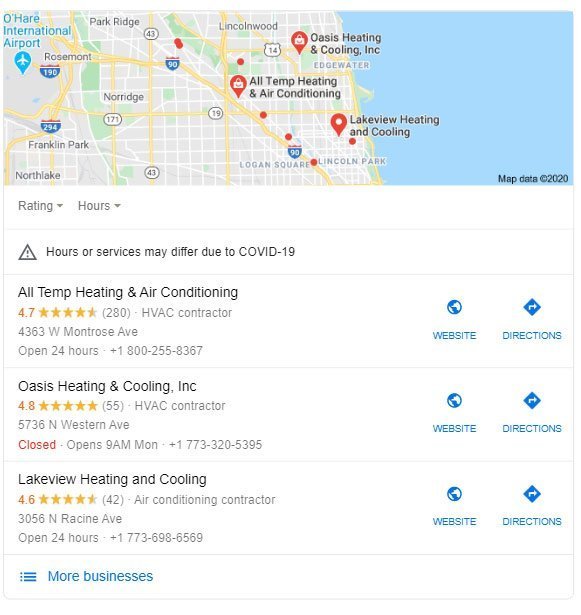This screenshot depicts a map interface, likely from MapQuest or a Garmin app, focusing on the Chicago Metropolitan area. Predominant locations include Lincolnwood, Norwich, Park Ridge, O'Hare International Airport, Franklin Park, North Lake, and Logan Square.

Highlighted on the map are several HVAC businesses, each marked with standout icons. Oasis Heating and Cooling Incorporated and All Temps Heating and Air Conditioning are flagged with red teardrop icons featuring shopping bags, signifying their commercial nature. Lakeview Heating and Cooling is marked with a similar red teardrop icon, but with a circle in the center instead of a shopping bag, indicating a different category.

Beneath the map, there is a section titled "Rating and Hours," warning that operating hours and services might vary due to COVID-19 precautions. The businesses are listed sequentially, starting with All Temps Heating and Air Conditioning, followed by Oasis Heating and Cooling, and ending with Lakeview Heating and Cooling. Each listing provides options for obtaining directions to the business or visiting their website, indicated by blue icons to the right of the business names.